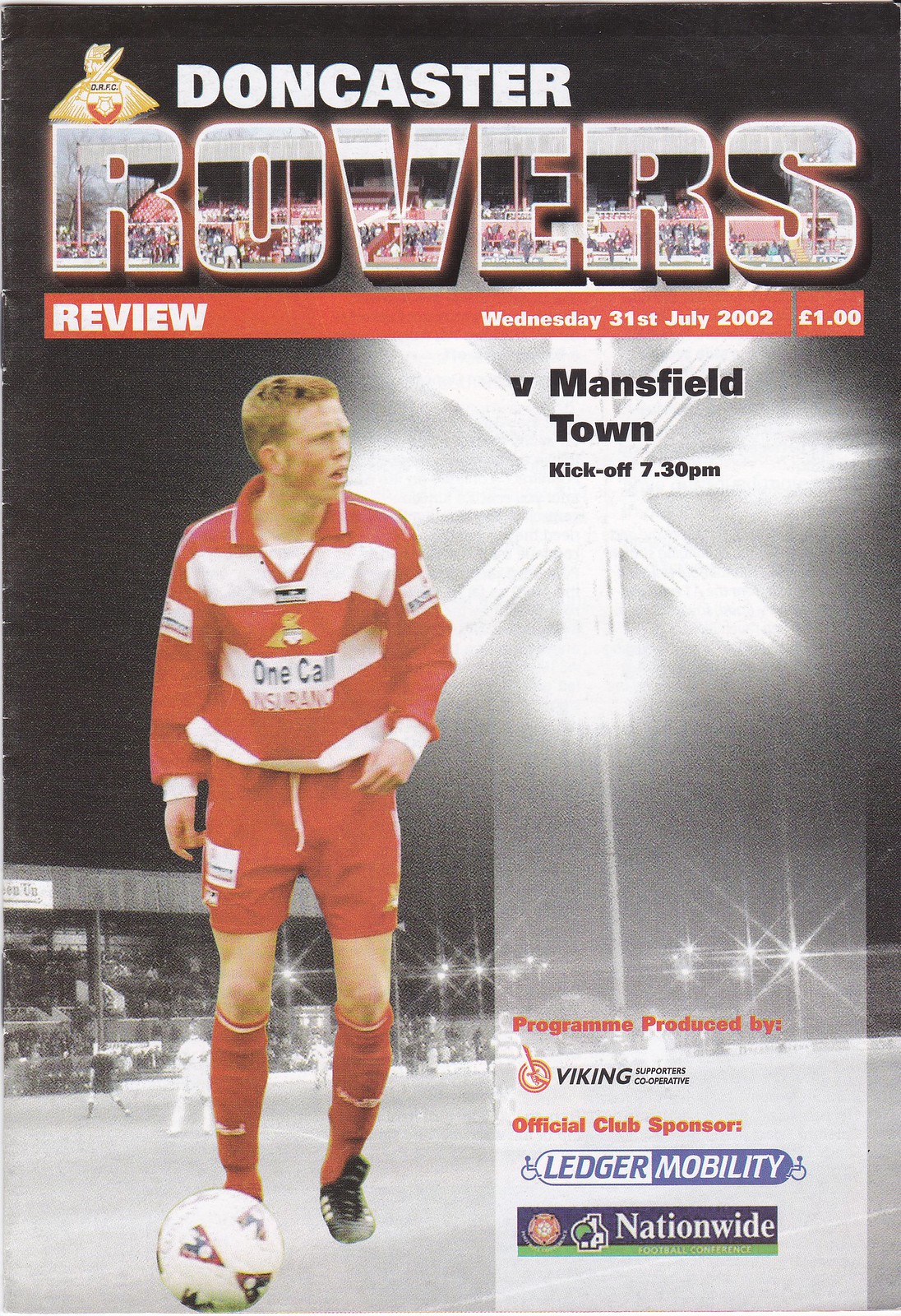The front page of this magazine-style flyer prominently features a bold header, "Doncaster Rovers," with the word "Rovers" adorned by imagery of a soccer audience or field. Below this title, a vibrant red banner states "Reviews," along with the publication date. Central to the layout is a dynamic image of a soccer player donning a red and white horizontally striped jersey, red shorts, red protective socks, and black shoes, with red hair matching the team's colors. In front of him lies a distinctive black and white soccer ball accented with red details. The player stands on a black and white depiction of a soccer field with spectators, while beams of bright light illuminate him from the field lights above and to the right. At the lower right corner, various sponsor listings, including Viking, official club sponsor, and Ledger Mobility Nationwide, are visible. The program details a match between Doncaster Rovers and Mansfield Town, with a kickoff time slated for 7:30 PM. The player's jersey features "One Call Insurance," adding to the array of sponsorships on this eye-catching cover.